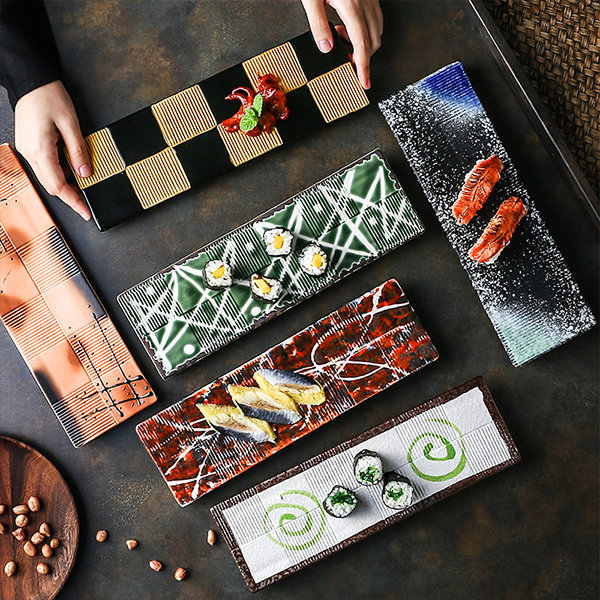This aerial-view photograph showcases a meticulously arranged selection of six long rectangular plates, each with distinct and vibrant designs, laid out on a dark, nearly black table. The plates are arranged in a checkerboard-like pattern and feature an assortment of colorful, potentially Japanese-style appetizers or sushi, though the exact dishes are hard to discern. 

Starting from the top left, one plate has a sophisticated black and white checkerboard motif, while another presents a striking green and white stripe pattern. The next plate boasts a distinctive orange and white striped design, followed by a plate with a subtle whitish-gray pattern. The fifth plate is a captivating dark black with gray, highlighted by specks of blue and white. The final plate on the bottom row is a vibrant red with white squiggly lines. 

Additionally, a round wooden bowl with a mix of seeds or nuts peeks out from the lower left corner of the image, adding an earthy contrast to the modern design of the plates. In the lower section of the photo, two hands are seen maneuvering one of the plates, suggesting an interaction with the food display. Overall, this visually arresting composition highlights an elegant and intriguing assortment of foods, inviting curiosity and appreciation for the artistry involved.